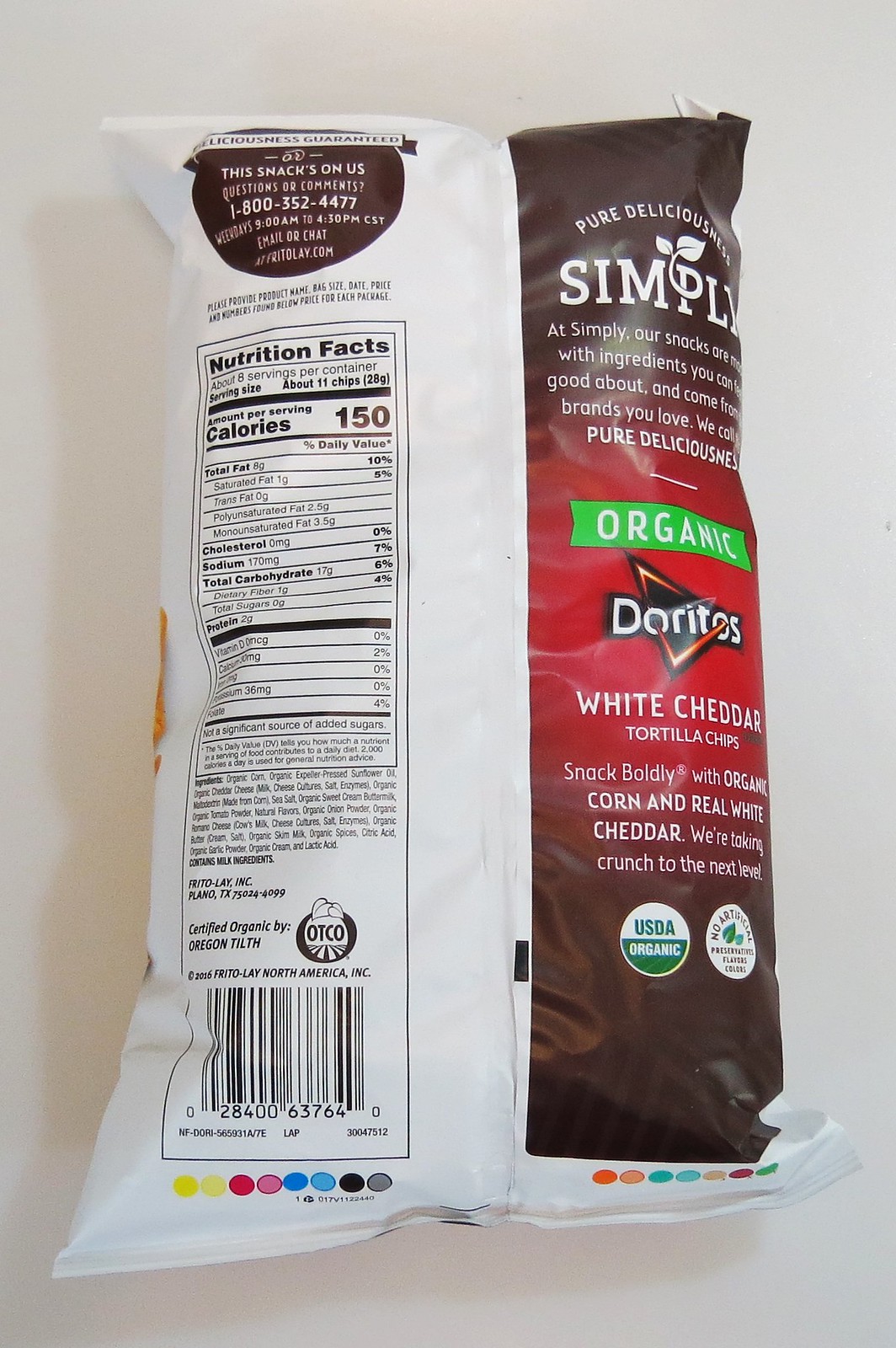This is a detailed close-up image of the backside of a bag of Organic Doritos, White Cheddar Tortilla Chips. The left side of the bag features a nutrition label indicating a serving size of 11 chips (28 grams), providing 150 calories. The nutritional facts are prominently displayed: 10% of the daily fat intake, 1 gram of saturated fats, no cholesterol, 7% of daily sodium, and 6% of total carbohydrate intake. Above the nutrition label is a bubble with a toll-free number for feedback if you are dissatisfied.

The right side of the bag has a visually appealing design with a red and brown ombre background, transitioning to a white panel. The top part of this section showcases the Doritos logo, which consists of a Doritos chip with the word "Doritos" over it, underneath a green banner with white "Organic" lettering. Below it, in bold font, it states "White Cheddar Tortilla Chips." Further down, there is a tagline encouraging you to "snack boldly with organic corn and real white cheddar," along with a statement reading, "At Simply, our snacks are made with ingredients you can feel good about and come from brands you love. We call this pure deliciousness."